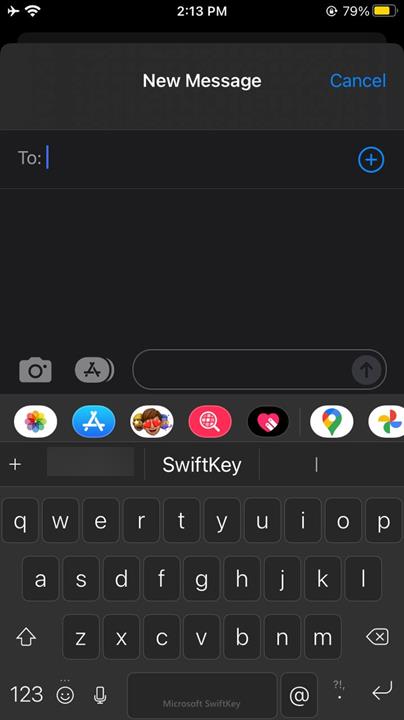The image is a screenshot of an iPhone in dark mode. The iPhone's interface elements confirm its identity. At the top-left corner, two white symbols are visible: one for airplane mode and another for Wi-Fi. Centrally aligned at the top is the time, showing 2:13 p.m., also in white. On the top-right corner, there's the portrait lock symbol indicating the screen orientation is locked. Adjacent to this, the battery percentage reads 79% and the battery icon is yellow, signifying that low power mode is activated.

The main screen displayed is for creating a new message. At the top, "New Message" is written in white, accompanied by a blue "Cancel" button. Beneath this, there's a white text box labeled "To" for entering recipient information, alongside a blue "+" button to add contacts. Below this are greyed-out camera and app buttons, followed by a cylindrical text box for typing the message, and a corresponding blue arrow send button.

Further down, there is an array of app icons including Photos, App Store, Emojis, Image Search, Touch Keys, Maps, among others. Immediately below the app icons, there is a "+" sign and an option for SwiftKey, providing alternative typing methods. At the bottommost part of the screen is the standard QWERTY keyboard in lowercase. This keyboard includes buttons for shift, delete, number and emoji switching, dictation, SwiftKey, spacebar, "@", period, and enter.